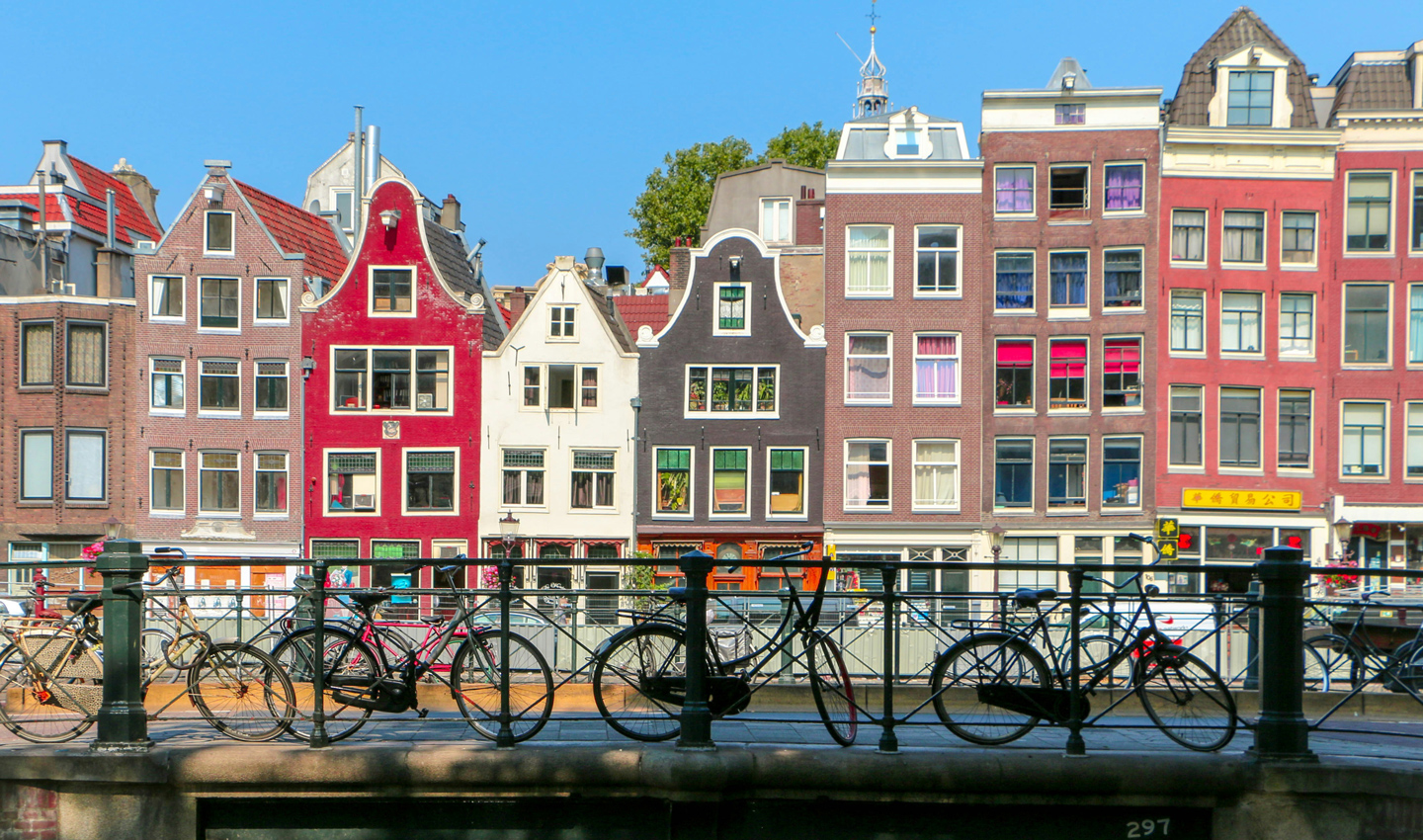This landscape-oriented color photograph captures a row of multi-story, connected townhouses lining a canal in Amsterdam, framed against a brilliant blue sky. The houses, ranging from three to five stories high, feature a variety of warm, muted tones including various shades of red brick, dark purple, light brown, and salmon-pink. Their roofs are equally diverse, with some arched and others pyramid-shaped, and include architectural details like bay windows and tower structures. Each building has windows that face the camera, bordered in shades of tan pink, light brown, and white. Notably, two buildings on the right have white roofs, one adorned with a cross and another with a window. In the foreground, a metal railing spans the width of the image, in front of which about six bicycles are leaned, silhouetted dramatically against the colorful backdrop of the townhouses. The water of the canal is light blue and partly visible just beyond the railing. The style of the photograph highlights representational realism, vividly capturing the characteristic charm of Amsterdam’s urban landscape.